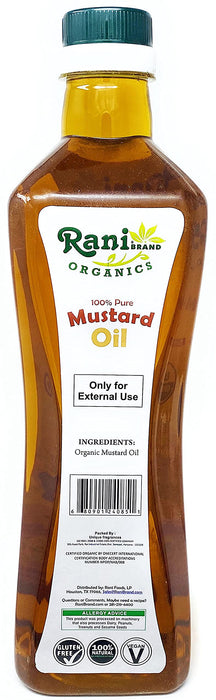The image depicts a tall, slender bottle of mustard oil with a distinctly rectangular shape that curves inward at the center, giving it an hourglass appearance. The bottle contains a golden-amber liquid and is capped with a dark green twist cap, underlined by a white and yellow band. The front label features a white background with the brand name "Rani Brand Organics" written prominently in green, accompanied by a yellow flower design. Below the brand name, "100% Pure Mustard Oil" is boldly printed in red and yellow font. There is also a black rectangle with "ONLY FOR EXTERNAL USE" clearly marked. Further down the label are various crucial details: an ingredients list in black font, a barcode, and three distinct logos indicating the product's gluten-free, 100% natural, and vegan certifications. The overall composition gives a clear view of a meticulously labeled, naturally sourced mustard oil product, perfectly suitable for online grocery shopping aesthetics.